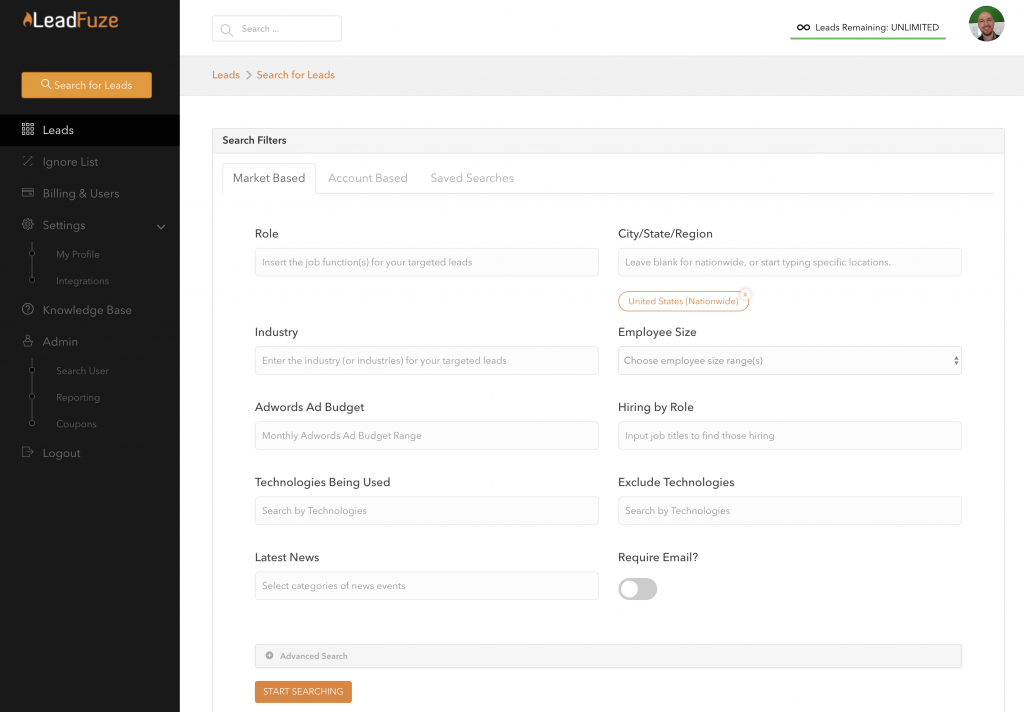The screenshot depicts a webpage from a platform called LeadFuse. The website's name is styled as one word with "Lead" in white and "Fuze" in orange. A black vertical navigation bar on the left features a list of options in gray font. The topmost option, highlighted with a heavier black shade and white text, is "Leads." The menu items are as follows: Search for Leads (with an orange button), Leads, Ignore List, Billing & Users, Settings, My Profile, Integrations, Knowledge Base, Admin, Search Users, Reporting, Coupons, and Log Out.

Adjacent to the navigation bar, at the top of the main section, there is a search bar labeled "Leads" with a downward-facing caret to its right. The phrase "Search for leads" is displayed in orange. Below the search bar, there is an infinity symbol indicating that the search capacity is unlimited. However, a green bar next to this symbol suggests the users might have already utilized some of their searches. 

Further down, the page presents a section titled "Search Filters" with the following categories: Market-based, Account-based, and Saved Searches. Currently, the "Market-based" section is expanded, revealing input fields for "Role," where users can insert job functions for their target leads, and "Industry," where users can specify the desired industry for their target leads. Additional fields include "AdWords Ad Budget," allowing users to define the monthly AdWords budget range for their target leads.